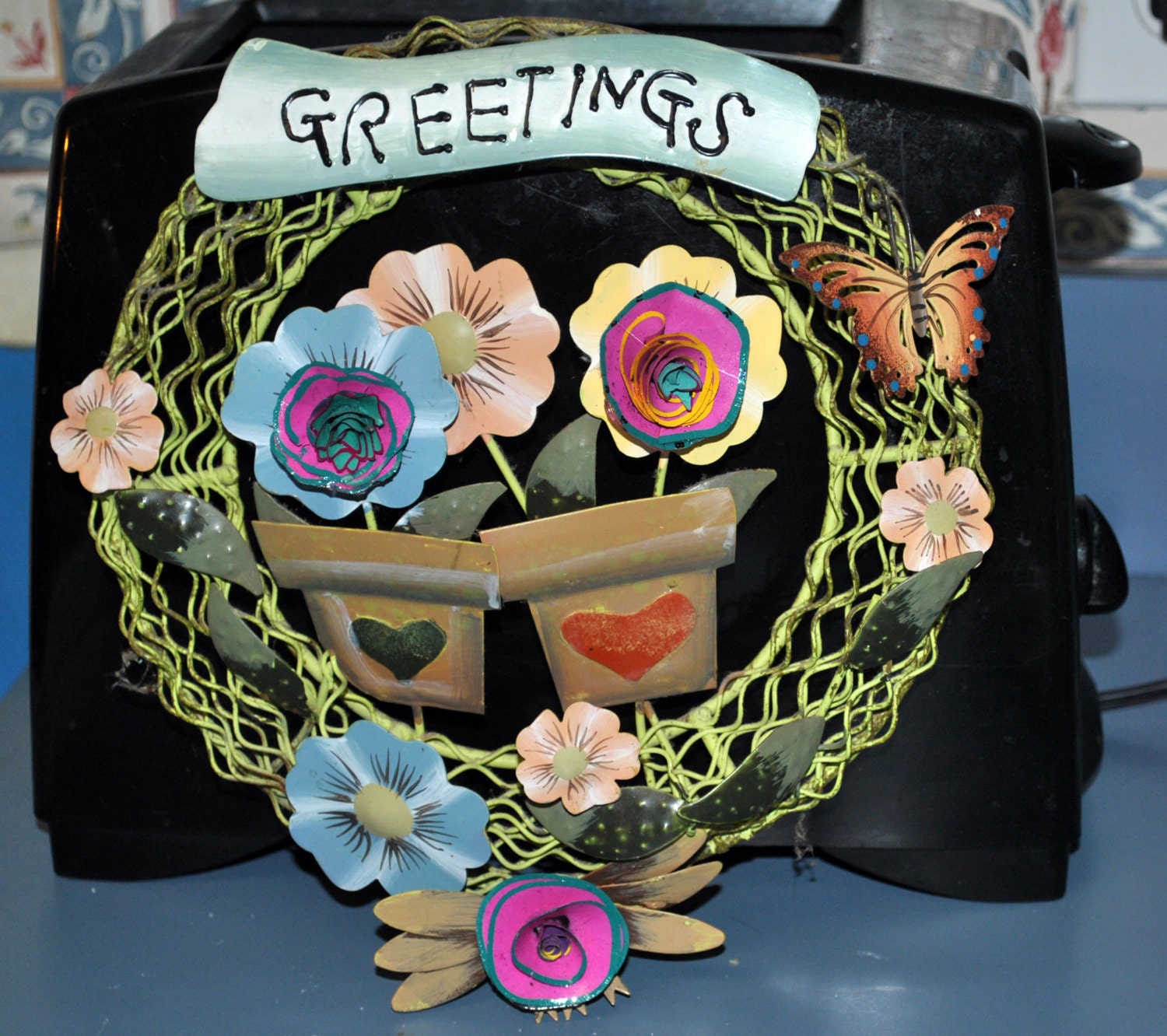The photograph features a meticulously crafted circular artwork composed of intertwining plant stems, roots, and sticks, forming a naturalistic base. This unique piece is adorned with an array of vibrant, artistic flowers held in custom, one-of-a-kind flower pots. At the apex of the artwork, a swooping sign spells out "Greetings" in paint that appears to have been artistically squeezed from a tube. Scattered throughout the piece are delicate butterflies and a variety of leaves, enhancing its organic and whimsical aesthetic. 

Set against this intricate backdrop of woody materials, the entire composition leans against a black toaster, the details of which—such as the adjustment knob, trigger, and electrical cord—are clearly visible on the right side of the image. The scene is anchored on a blue-green countertop, with additional tiles glimpsed in the background, providing a snapshot of a domestic setting. This detailed, floral-themed artwork, which would typically be displayed on a door or wall, finds an unusual temporary resting place, adding an unexpected layer of charm and quirkiness to the photograph.